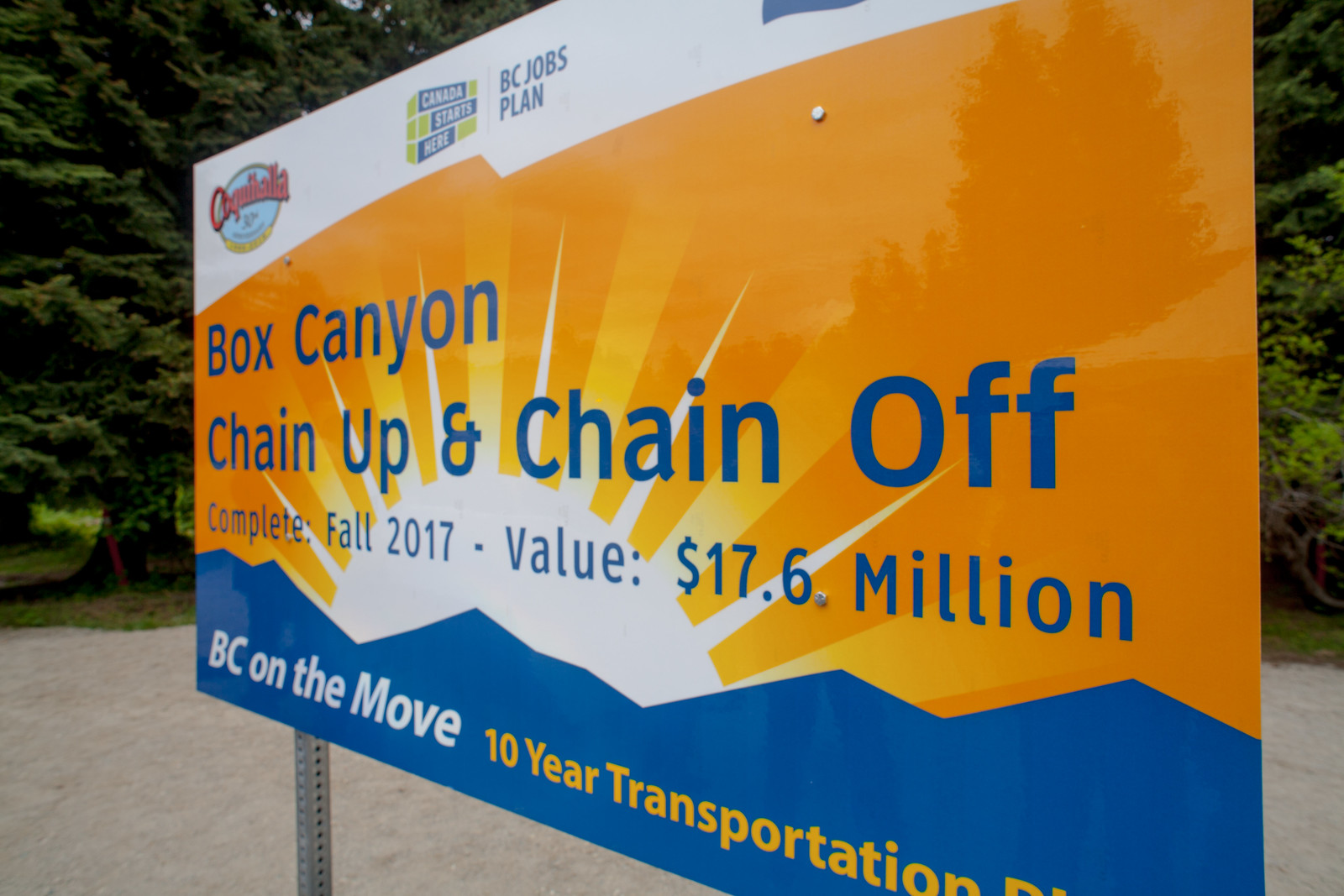This is a color landscape orientation photograph of an outdoor billboard sign located in a sandy area, possibly a beach, with green trees in the background. The sign, which stands on two steel posts, describes a development project slated for completion in Fall 2017 with a value of 17.6 million dollars. The sign is prominently divided into several sections: 

- The top section features three small logos on a white background with "BC Jobs Plan" written next to them.
- The main central section is a bold orange with a white rising sun graphic over a blue mountain range at the bottom. Here, the blue lettering reads "Box Canyon Chain Up and Chain Off" followed by "Complete: Fall 2017" and "Value: 17.6 million dollars."
- The bottom section is blue with white and gold text, showing "BC on the Move" and "10-Year Transportation." This part also has design elements resembling water waves.

The photograph highlights a perspective angle view of the sign against a backdrop of greenery and beige sand, underscoring its detailed design and informational content.